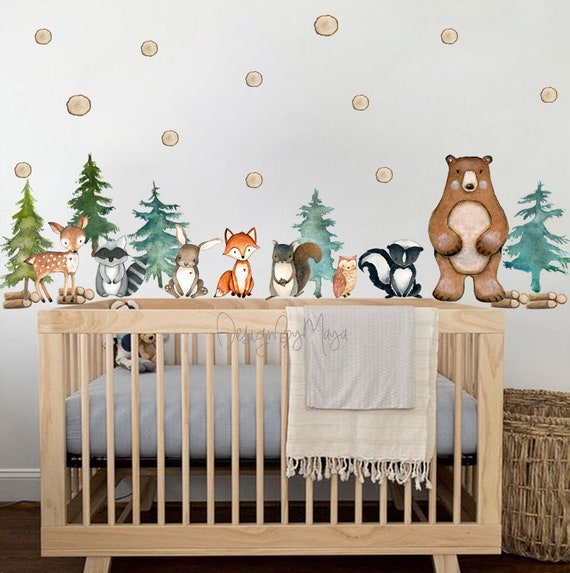This detailed indoor color photograph captures a close-up view of a nursery centered on a wooden crib, which appears to be handcrafted from light-colored, possibly unfinished maple or light pine wood. The crib's slats are prominently featured, and inside, a neatly arranged blue mattress sits. Draped over the crib's railing are two folded blankets: a larger tan blanket with fringes and a smaller light blue blanket atop it. The nursery wall behind the crib is adorned with an endearing mural of cartoon forest animals, aligned and facing the camera, including a small deer, raccoon, rabbit, fox, squirrel, owl, skunk, and a slightly larger bear. Above these animals, whimsical brown polka dots are scattered. Positioned on the floor to the right of the crib is a large, brown wicker basket. The flooring itself is a dark brown hue, adding contrast to the scene. Additionally, within the crib are two small stuffed animals, one appearing to be a teddy bear. The photograph features a watermark signature of the photographer positioned centrally, contributing to its overall symmetry, subtly disrupted by the basket on the right.